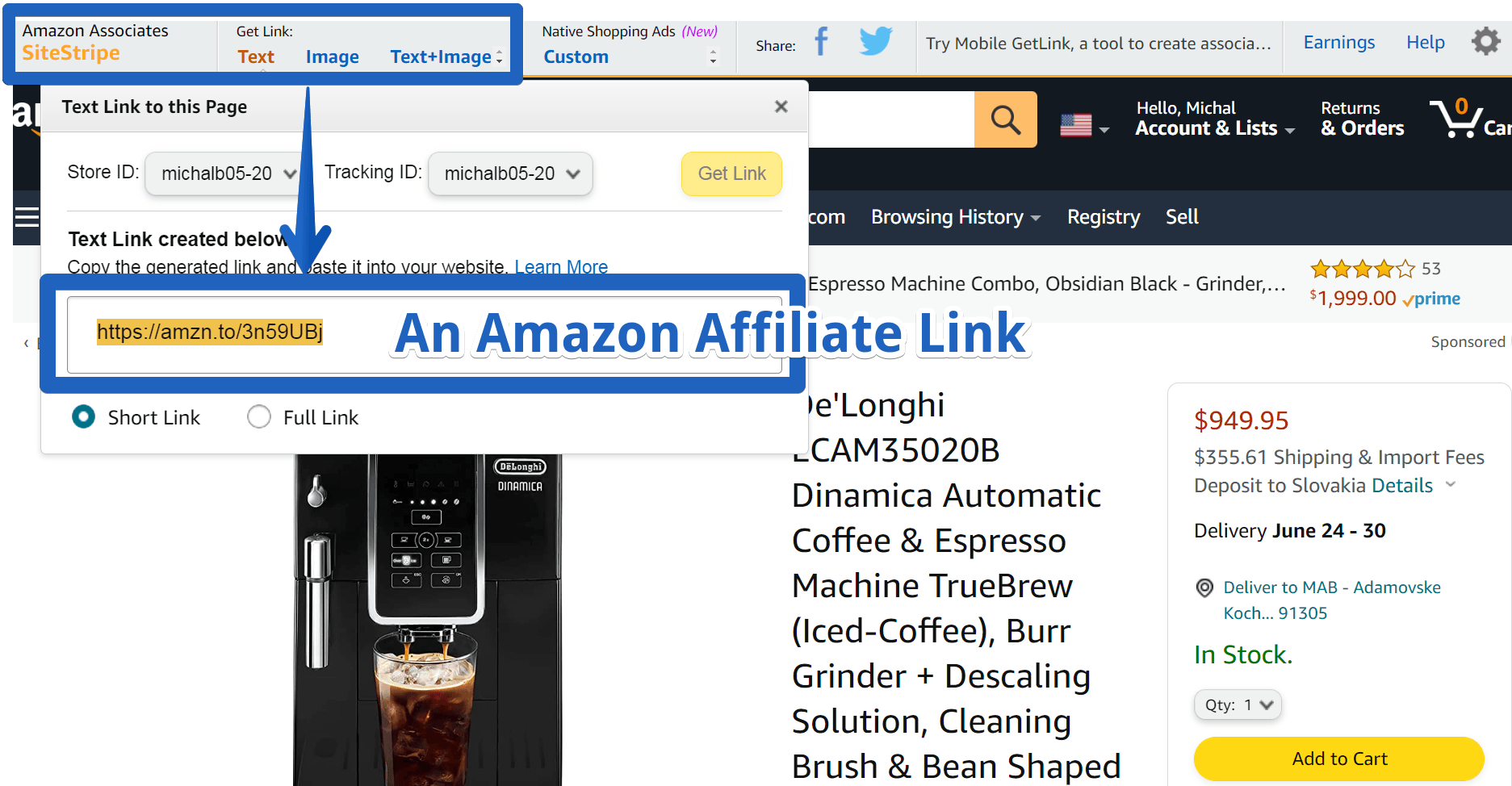The image depicts a webpage specifically designed for Amazon Associates, featuring a detailed interface for creating affiliate links. 

At the top of the page, there is a blue square highlighting the text "Amazon Associates" in black print. Adjacent to it, "SiteStripe" is displayed with both S's capitalized and in orange text. Below this, options to "Get Link" are presented, showing choices for "Text" in a darker orange, and "Image" and "Text+Image" in blue text. 

A downward-pointing arrow leads to a larger banner with a blue border, displaying an affiliate link "HTTPS://AMZN.TO/3N59UBJ" labeled as "Amazon Affiliate link." Beneath this, there's an option between "Short link" and "Full link," with "Short link" being selected.

Further up again, a purple text titled "Native Shopping Ads (new)" is visible, followed by a blue "Custom" link. The interface also provides options to "Share" on "Facebook" or "Twitter," with additional features like "Try mobile," "Get link," "A tool to create associate...," "Earnings," and "Help."

The middle section of the page explains the creation of text links, indicating with "Text link to this page," "Door ID," and "Text link created below." Users are instructed to "Copy the generated link and paste it to your website," with an additional option to "Learn more."

This organized and color-coded layout helps Amazon affiliates easily create and manage links, facilitating a seamless integration into their websites.